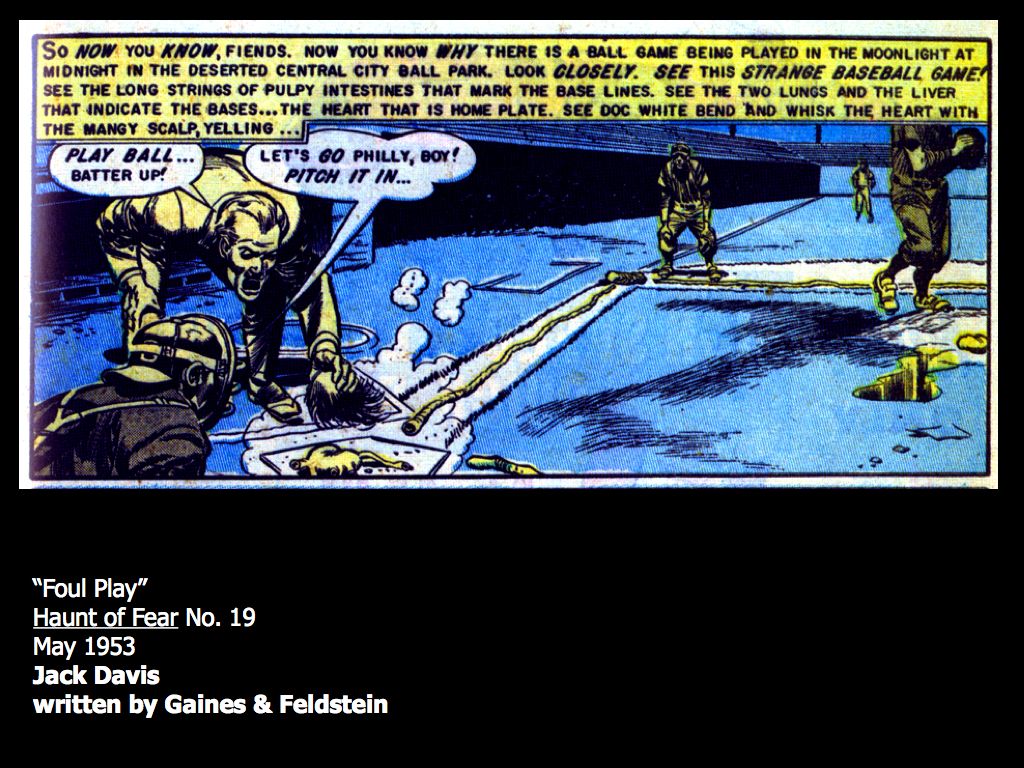The image is an eerie comic strip with a black background and a detailed border outlined in white. At the bottom right-hand corner, it reads "Foul Play (Haunt of Fear No. 19)" with "Haunt of Fear" underlined. Below this, the text "May 1953, Jack Davis, written by Gaines and Feldstein" is displayed. The comic portrays a ghoulish baseball game being played in the moonlit, deserted Central City ballpark at midnight. The field is marked by grotesque, anatomical elements: pulpy intestines form the baselines, and organs such as lungs, a liver, and a heart serve as bases and home plate. Doc White is seen bending over the heart, brandishing a mangled scalpel and yelling "Play ball!" and "Batter up! Let's go, Billy boy, pitch it in." The characters in the scene are drawn in a dark blue, white, and yellow color palette to suggest a night scene. An umpire stands in black attire with yellow headgear, while the crowd stand appears in black and blue. Above the scene, the text "So now you know, fiends. Now you know why there is a ball game being played in the moonlight at midnight in the deserted Central City ballpark" sets the eerie tone of the strip.